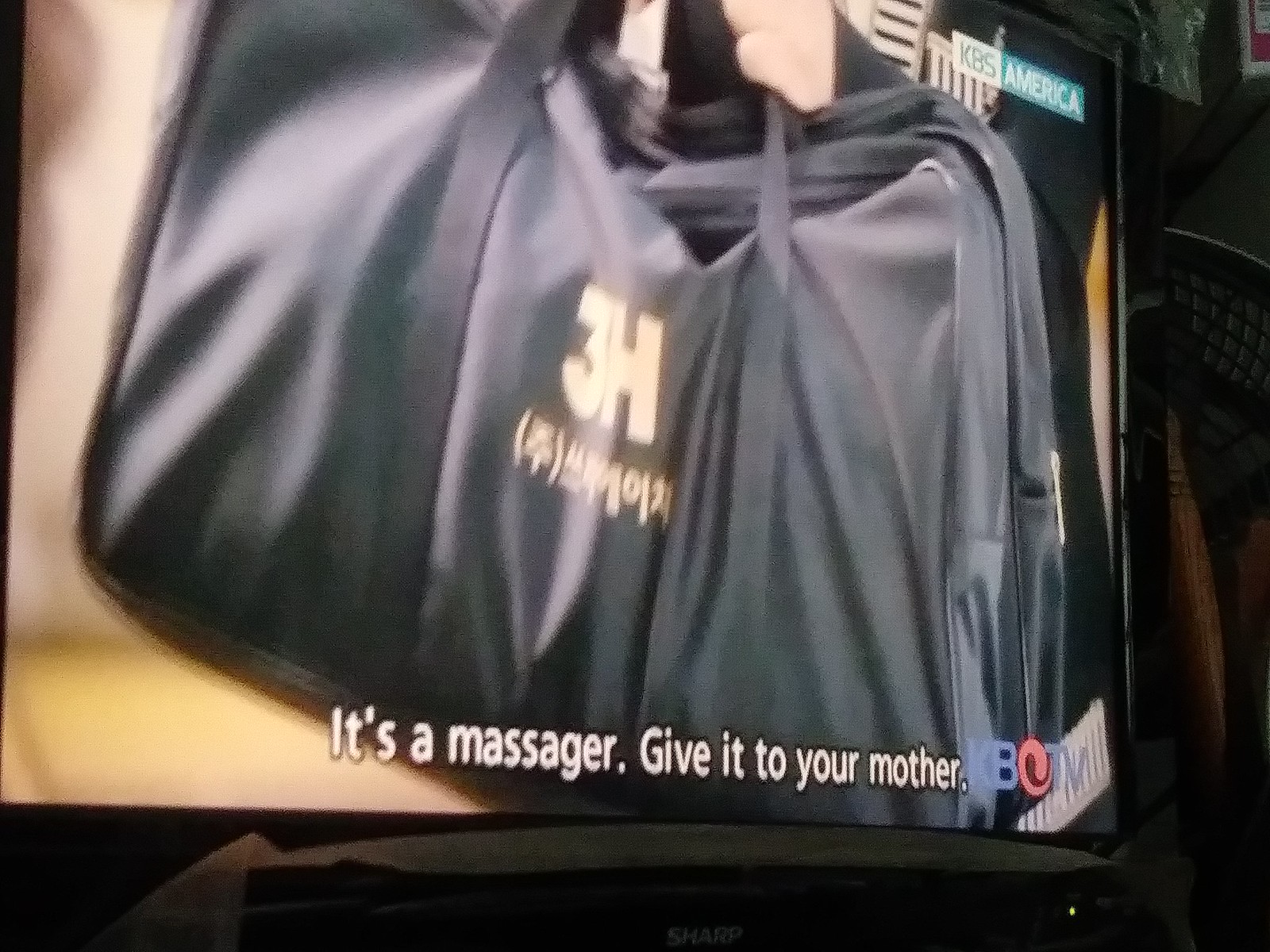The image is a photograph of a television screen displaying a black, flexible carrying bag with the logo "3H" printed in gold at the center front. Below the 3H logo, there are some Korean characters that are somewhat blurry and hard to decipher. The television screen also has closed captioning in an off-white sans-serif font at the bottom, showing the text: "It's a massager, give it to your mother." At the bottom right corner of the screen, there is a logo indicating the TV channel: "KBO TV," where the letters "KB" and "TV" are in blue, and the "O" is styled as a red swirl similar to an emblem seen on the Korean flag. Additionally, there's another smaller sign in the top right corner of the screen stating "KBS America," divided into two sections with "KBS" written in turquoise on a white background and "America" written in white on a turquoise background. The television itself has a black frame, and in the dark background to the right, there's a faint outline of what appears to be a laundry basket.